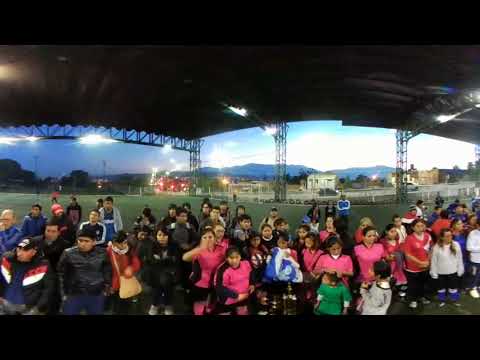In an open-air sporting facility, captured during the evening, a large group of people stands attentively under a broad industrial tent supported by several metal pillars. The sky above is a dark blue, peppered with white clouds, hinting at the end of the day. The crowd is predominantly female on the left and center, many wearing pink jerseys, while the right side consists mostly of males in red or burgundy jerseys. Everyone's gaze is fixed forward, likely watching a live sporting event or a game on a large screen. In the backdrop, a vast field, either grass or astroturf, extends into the background, with a couple of people visible on it. Beyond the field, a scattering of buildings lines a road where a few cars are seen moving, and in the far distance, a range of mountains forms a serene horizon. Street lamps are beginning to illuminate the scene, adding to the tranquil ambiance as the day transitions into night.